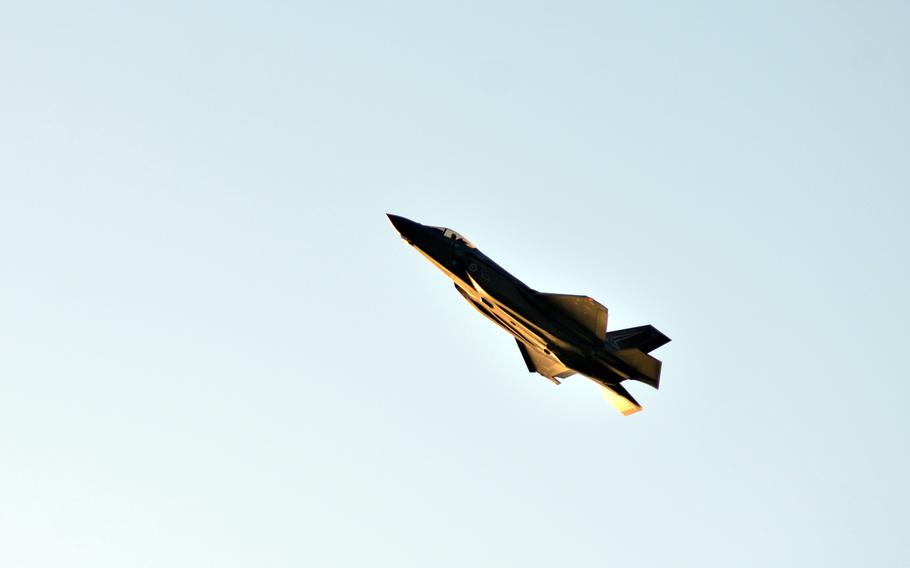The photograph captures an F-35 fighter jet climbing steeply into the sky, angled towards the upper left-hand side of the image. The background features a pale greenish-blue sky that gradually becomes a solid light blue, indicative of an outdoor daytime scene. The jet, with a modern, stealthy design, is primarily silhouetted against the sky, but the underbelly is illuminated by sunlight, casting a yellowish-brown tone. The top portion of the aircraft remains in shadow, making its grey, silverish, or potentially even black coloration hard to discern. The jet showcases a sharp nose, a cockpit with a visible pilot's head, and distinctive tail structures consisting of a vertical fin and two horizontal fins. There's also a red light visible at the tip of one wing, adding to the detailed features of this formidable, Mach 2-capable aircraft. The entirety of the scene is subtly shadowed, with the light source coming from below and to the left, emphasizing the jet's ascent and giving depth to its appearance.